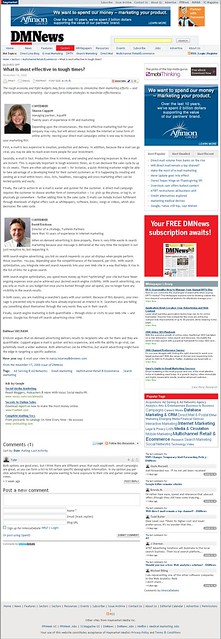This image depicts a screenshot of an article captured on a mobile device. The article's layout is predominantly white with black text. A blue banner featuring a sun icon and what appears to be the word "Affirmation" spans across the top, although the text is difficult to discern due to the distance. The header prominently displays "DM News" in large, bold black letters. On the right side, a yellow-highlighted search bar is visible. Just below the header are several tabs, with one tab encased in a red box, although the specific labels on these tabs are not readable. The highlighted tab reads, "Your free DM News subscription awaits," with a red background indicating a newsletter notification. The article includes two photographs: one of a woman with short blonde hair wearing a black shirt and smiling, and another of a man with short gray hair, wearing a button-up white shirt and black tie, also smiling.